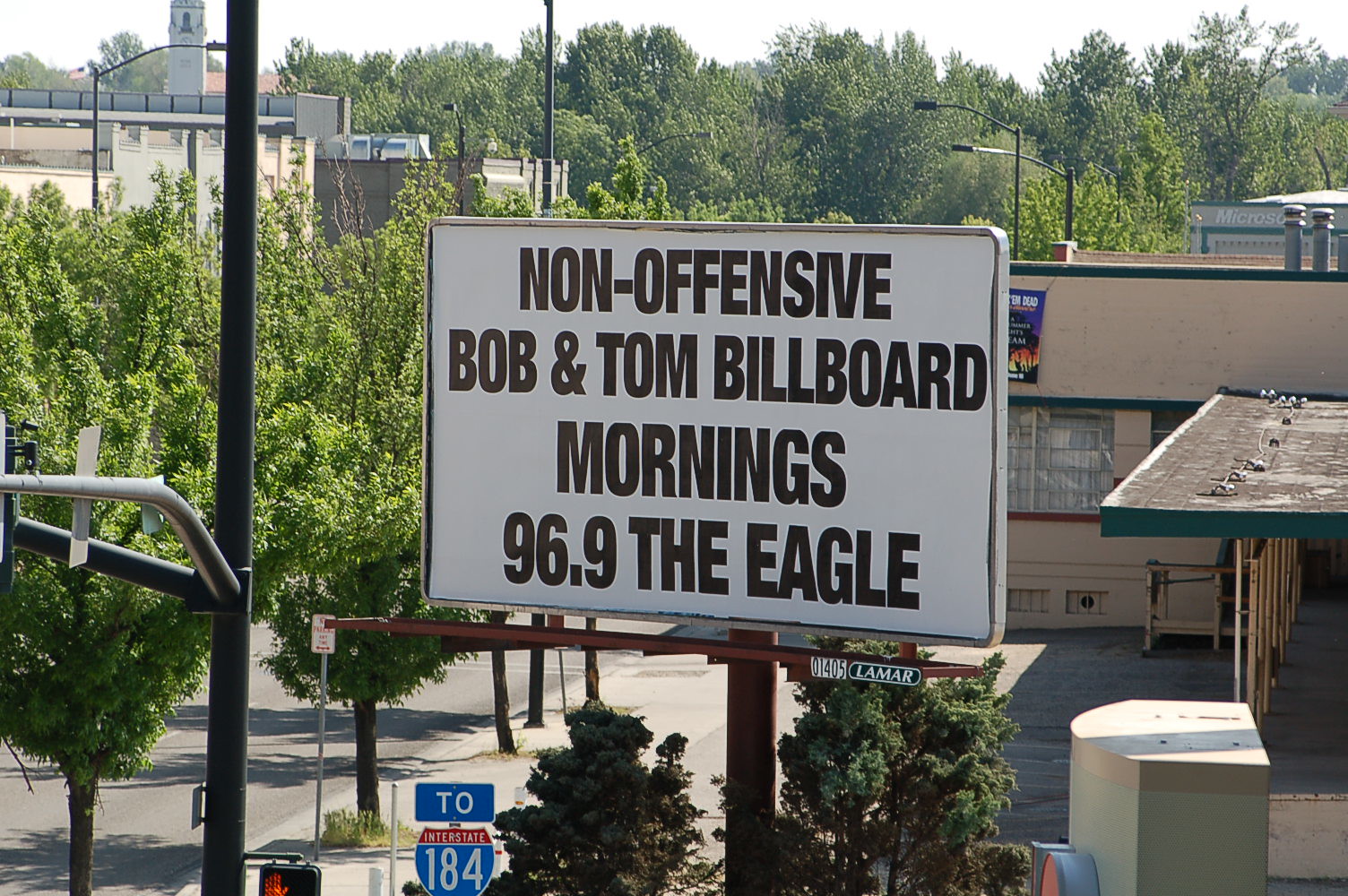This angled photograph captures a small, square billboard in a semi-suburban area. The billboard, set against a white background with a silver base, displays black uppercase text that reads "Non-offensive Bob & Tom Billboard Mornings 96.9 The Eagle." The frame of the billboard includes the label "Lamar 01405." The billboard, supported by a short, round brown metal pole, towers just above a nearby tree to the right and is barely taller than a building in the background, which features a green bordered awning that appears warped. 

The background reveals a mix of trees and buildings, including a gray building with green trim that seems to have the word "Microsoft" in white letters across the top. Below the billboard, a blue interstate sign indicates Interstate 184, with 'Interstate' written in red and '184' in blue, accompanied by a street sign reading "2." There's also a partially visible pedestrian crosswalk signal displaying a red hand. In the bottom left corner of the photo, a crosswalk signal and another street sign that states "No Parking At Any Time" can be seen. The overall scene suggests a blend of natural elements and urban infrastructure.